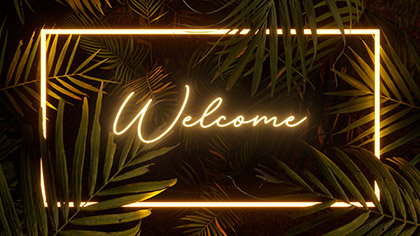The image features the word "Welcome" written in glowing, cursive neon text, prominently centered against a dark red, moody background. Surrounding the "Welcome" sign is a rectangular neon light that forms a shining frame, giving the whole image a radiant, almost ethereal quality. Palm fronds, both in front of and behind the neon frame, stretch in from every direction, creating a circular pattern around the text. The neon lights of the sign and the frame illuminate these palm fronds, adding depth and intrigue to the composition. The overall scene resembles a high-contrast, Instagram-worthy photograph and evokes a welcoming yet mysterious atmosphere.